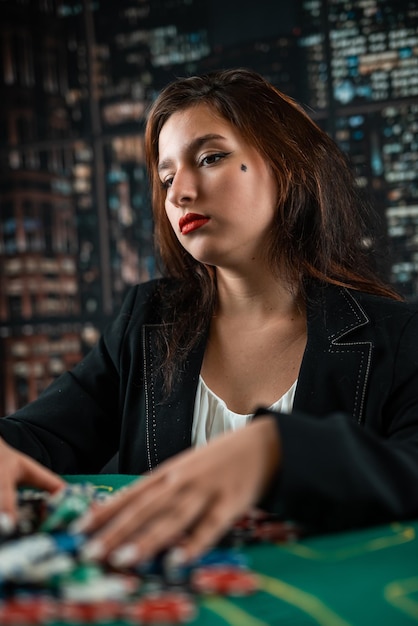The image features a Caucasian woman with medium brown, shoulder-length hair, seated in front of a multi-paned window showcasing a backdrop of various lit, but blurred, skyscrapers. A noticeable black beauty mark adorns her left cheek. She is wearing mascara, white eyeshadow, and red lipstick, complementing her black denim jacket over a white blouse. In the foreground, her hands, slightly blurred, display white nail polish as she appears to either hold or slide a collection of multi-colored poker chips (white, red, and blue) on what looks like a green poker table. The scene suggests she is engaged in a poker game within a high-rise building.